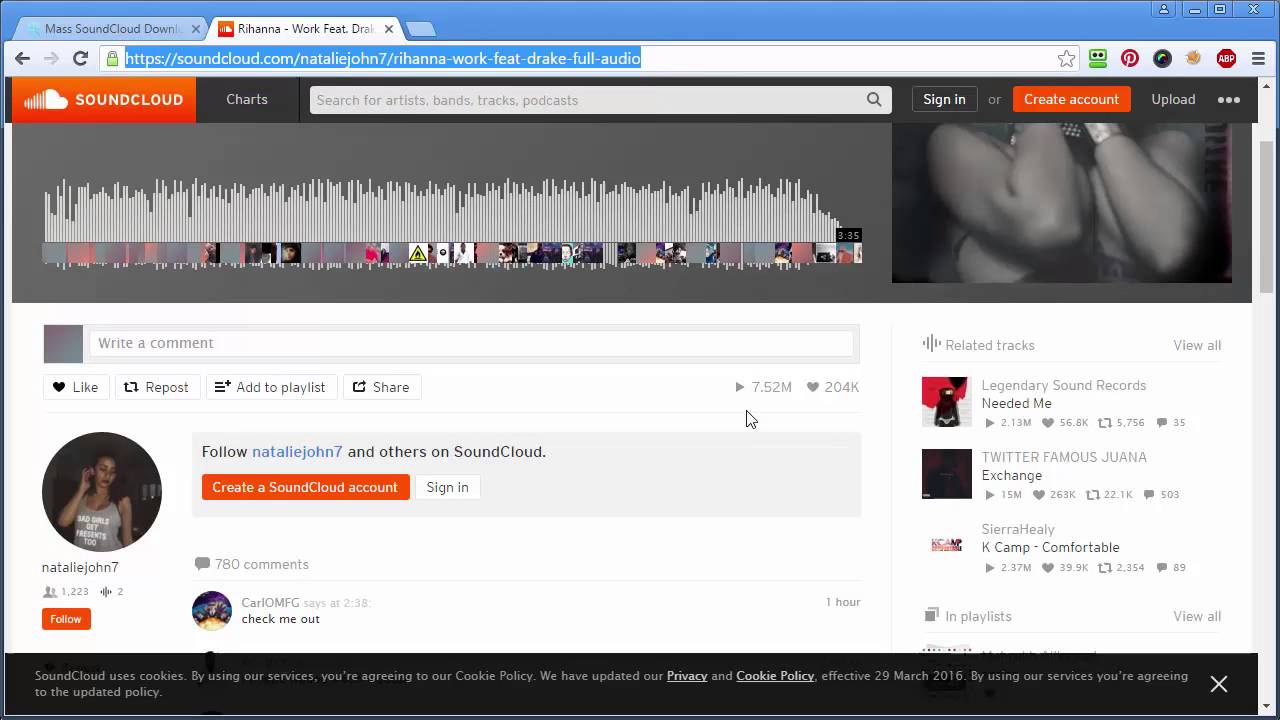The desktop screenshot showcases a web browser on a Microsoft computer, although the specific browser cannot be identified. The user has two tabs open. The first tab appears to be a tool for mass downloading from SoundCloud, suggesting potentially improper use of downloaders. The second tab, which is currently active, displays a SoundCloud page for Rihanna's song "Work," featuring Drake.

The URL in the selected tab is: `https://soundcloud.com/nataliejohn7/rihanna-work-feat-drake-full-audio`. The interface includes the browser's back, forward, and refresh buttons, as well as indicators that the site is secure (HTTPS). Bookmark icons include a green robot, Pinterest, a pie chart-like icon with a section of a rainbow, and ABP for AdBlock, along with a hammer icon for more options.

In the SoundCloud interface, there's an orange header with a white cloud logo that looks like it's fading. Users can navigate to Charts, search for various media types, sign in or create an account, upload content, and access more options via three dots.

The main content area shows the page is heavily interacted with: the track has been played 7.52 million times, "hearted" by 240,000 users, and the artist Natalie John has 1,223 followers with only two tracks released. There are 780 comments, including one from a user named Carl saying "OMG" at the 2:38 mark, posted an hour ago.

Adjacent to the comments section, related tracks are highlighted with their respective statistics:
- **Needed Me by Legendary Sound Records**: 2.13 million plays, 56K likes, 5,756 shares, 35 comments.
- **Joanna Exchange by Twitter Famous**: 15 million plays, 263K likes, 22.1K shares, 503 comments.
- **Comfortable by Sierra Healy & K Camp**: 2.37 million plays, 39.9K likes, 2,354 shares, 89 comments.

At the bottom, the page notes SoundCloud’s cookie policy update effective March 29, 2016, indicating that the user agrees to this policy by using the site, with an option to close the notice.

Overall, the screenshot provides a comprehensive view of user interaction with SoundCloud, showcasing extensive user engagement with the "Work" track and presenting related content with detailed statistics.